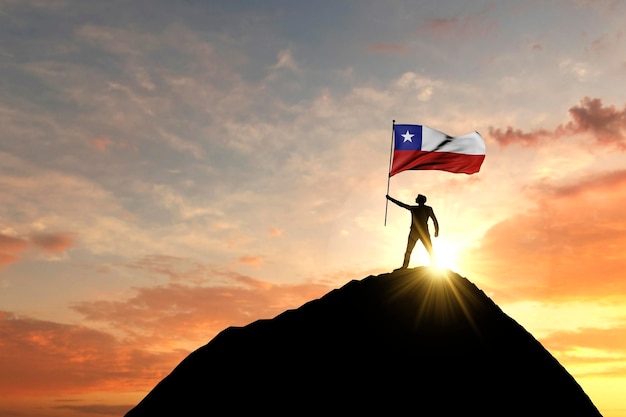In this captivating image, a silhouetted figure stands triumphantly atop a mountaintop, holding a flag high against the backdrop of a glowing sky. This striking flag, identified by some as potentially Chilean or Puerto Rican, features a blue square with a prominent white star, a white stripe adjacent to the square, and a broad red stripe beneath. The scene is bathed in the warm hues of a transitioning sky, with a peachy-yellow glow from the sunset enveloping the background. Wispy white clouds and touches of pink adorn the upper sky, while deeper shades of purple mix with bright and dark clouds lower down, enhancing the dramatic atmosphere. The sun, positioned near the mountaintop, casts golden rays that illuminate the landscape, creating an inspiring silhouette of the figure and the flag.